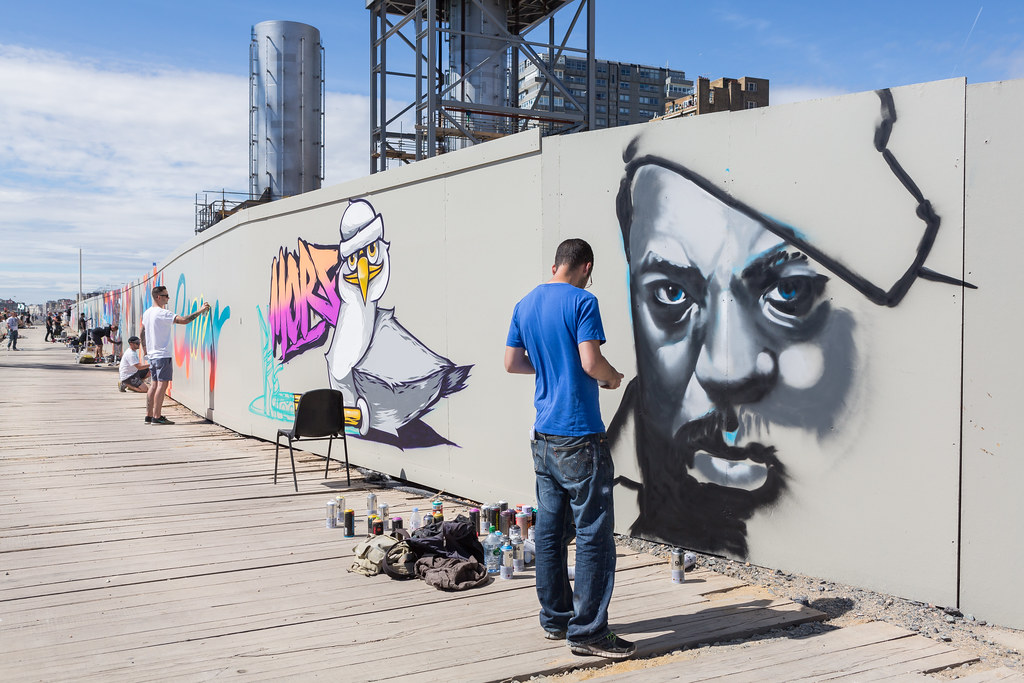This photograph captures a vibrant outdoor art exhibition on a boardwalk set against a backdrop of industrial factory infrastructure. The sun is shining brightly, illuminating the lively scene where diverse groups of people engage in creative graffiti artistry. The boardwalk, with its wooden panels, leads our eyes along a long, blank gray wall divided into sections for each artist.

In the foreground, a young man with pale skin, black hair, blue jeans, and a blue shirt stands next to an array of spray cans, intently working on a striking black and white portrait of a black man. This artist, possibly European, methodically details the half-completed face against the gray wall.

Adjacent to him, another painting bursts with color—vibrant orange and pink graffiti spelling out "Morf," with the accompanying image of a large white bird with a gray body. A chair sits in front of this artwork, yet its creator is absent from the frame.

As the scene extends into the background, it becomes harder to discern the individual artworks, but the wall is lined with more people actively painting. The artists, mostly men with varying olive and pale complexions, contribute to the dynamic, evolving mural under a light blue sky scattered with clouds. The bustling, creative atmosphere suggests a location reminiscent of a European setting, where community and art seamlessly blend together.